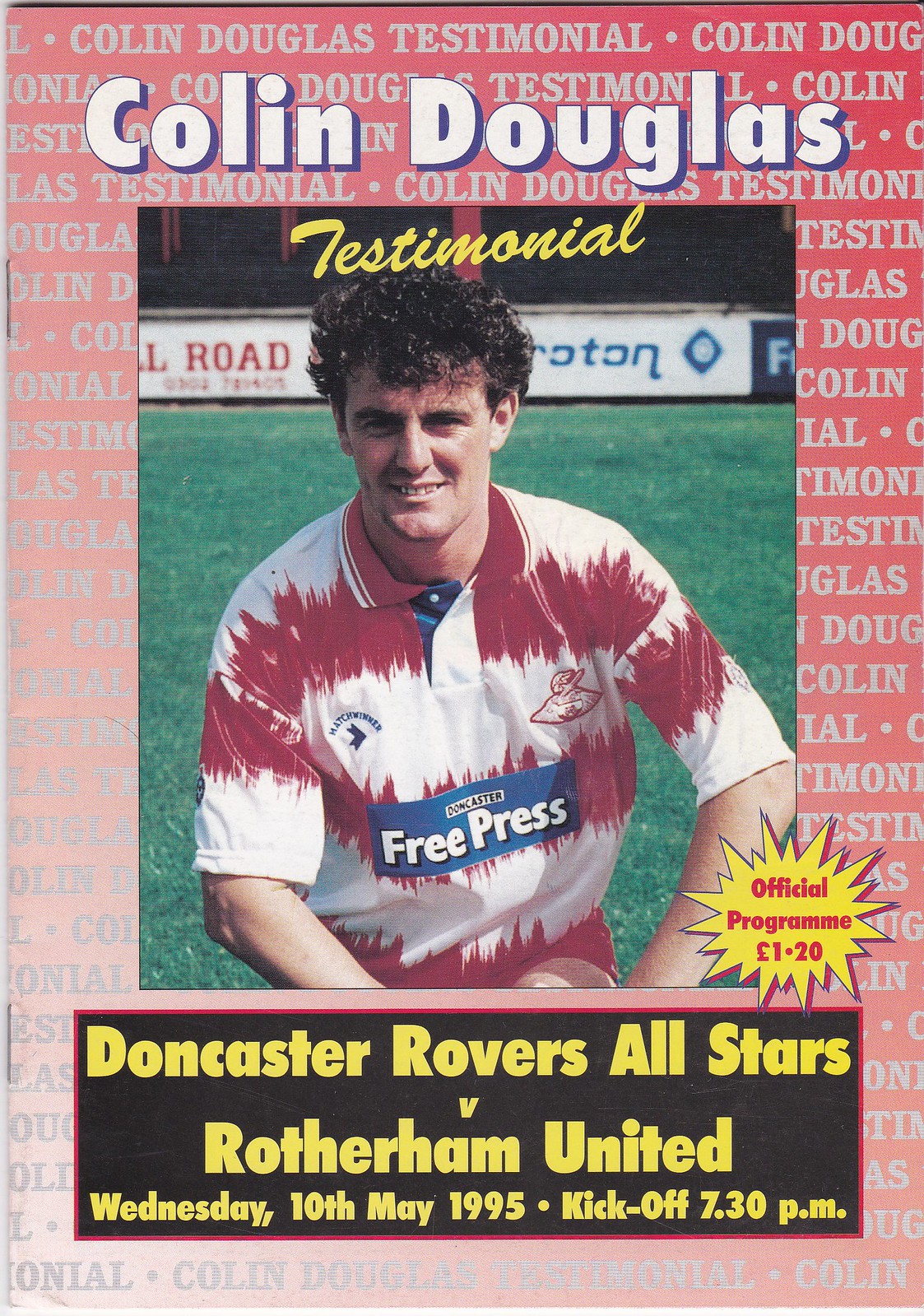This image displays a detailed cover of a football magazine, prominently featuring Colin Douglas, an English footballer, who is captured standing and looking directly at the camera in a grassy field with advertisement-covered walls in the background. Douglas is wearing a red and white striped shirt, and he has curly hair. The magazine appears to be from an English football club, likely associated with the Doncaster Rovers. The title "Colin Douglas" is at the top, with "testimonial" written in yellow text over a pink border against a brown background. The central focus of the cover is Colin Douglas's testimonial match, with details "Doncaster Rovers All-Stars vs. Rotherham United, Wednesday, 10th May 1995, Kickoff 7.30pm" written in yellow. There is also a small promotional graphic in the bottom right corner stating "Official Program 1.20 euro," designed as an exploding star. The colors of the magazine include red, pink, grey, white, green, blue, and black. The scene seems to be set outdoors during the day.